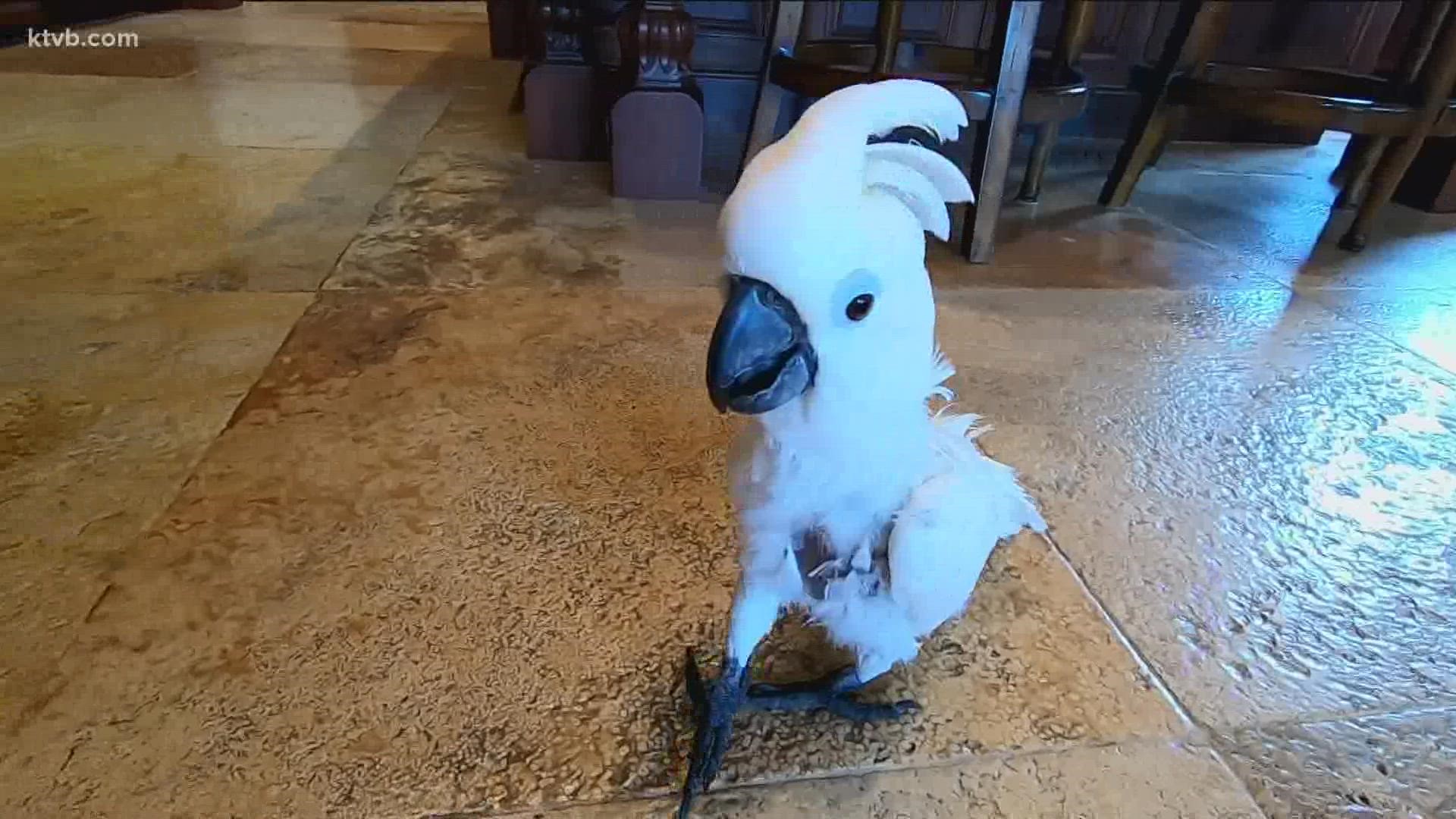The photograph captures an exotic white bird, possibly a cockatiel or a parrot, distinguished by its vivid black beak, black legs, and a striking feathered crown atop its head. The bird is situated on a brown ceramic or stone tile floor, adding a rustic charm to the indoor setting. In the background, there are the legs of wooden stools and a dark brown, wooden-paneled wall with matching baseboards, indicating it might be in a kitchen or dining area. The overall ambiance suggests a cozy, domestic environment where the bird appears free to roam. The bird's posture, with one foot slightly in front of the other, gives an impression as if it might be dancing. Adding a subtle detail to the image, in the upper left corner, small white text reads "ktvb.com."